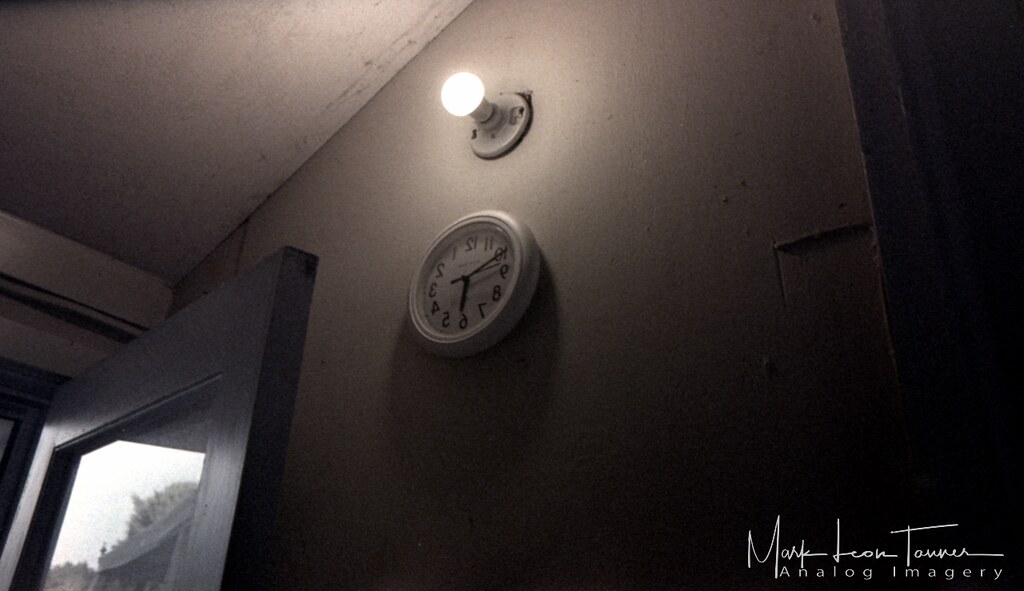This photo depicts a hallway featuring a striking mirrored or reversed perspective. Central to the composition is a clock mounted on a plain white wall, but the clock's numbers appear backwards, as if reflected in a mirror. Above the clock, there is an uncovered light bulb protruding from the wall. To the left, an open wooden door with a glass panel reveals a reflection of trees and bushes outside, hinting at daytime. The right side of the image fades into darkness. In the lower corner, the photographer's name, "Mark Leon Tanner," is signed in a stylized script, with the words "Analog Imagery" printed below in regular text.